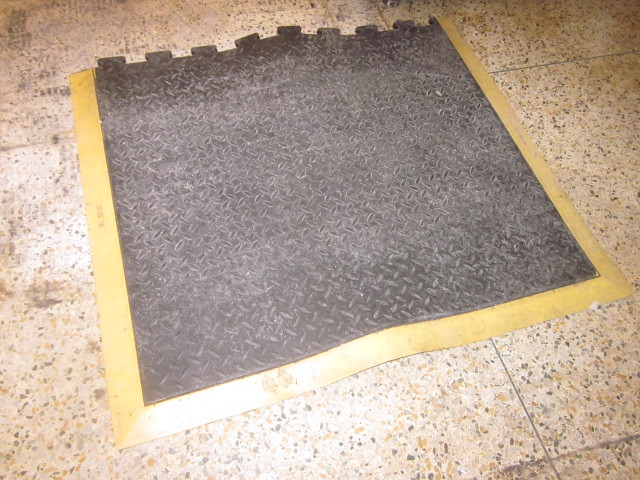This photograph features a large mat, prominently occupying most of the frame, set upon a floor of large square tiles. The tiles appear to be made of laminate and have a beige base color with flecks of gray and tan, resembling stone. The mat itself serves both decorative and functional purposes, likely intended for kitchen or industrial use. It has a textured surface characterized by a gray herringbone pattern in the center, showing signs of wear with swatches of white. The edges of the mat are bordered by a yellow-golden strip, which contrasts with the darker center. The mat’s sides are designed to interlock with additional sections, suggesting that it can be expanded to cover a larger area. This versatile and robust mat may be made of rubber or a similar durable material, and its placement on the patterned laminate flooring creates an intriguing visual juxtaposition.